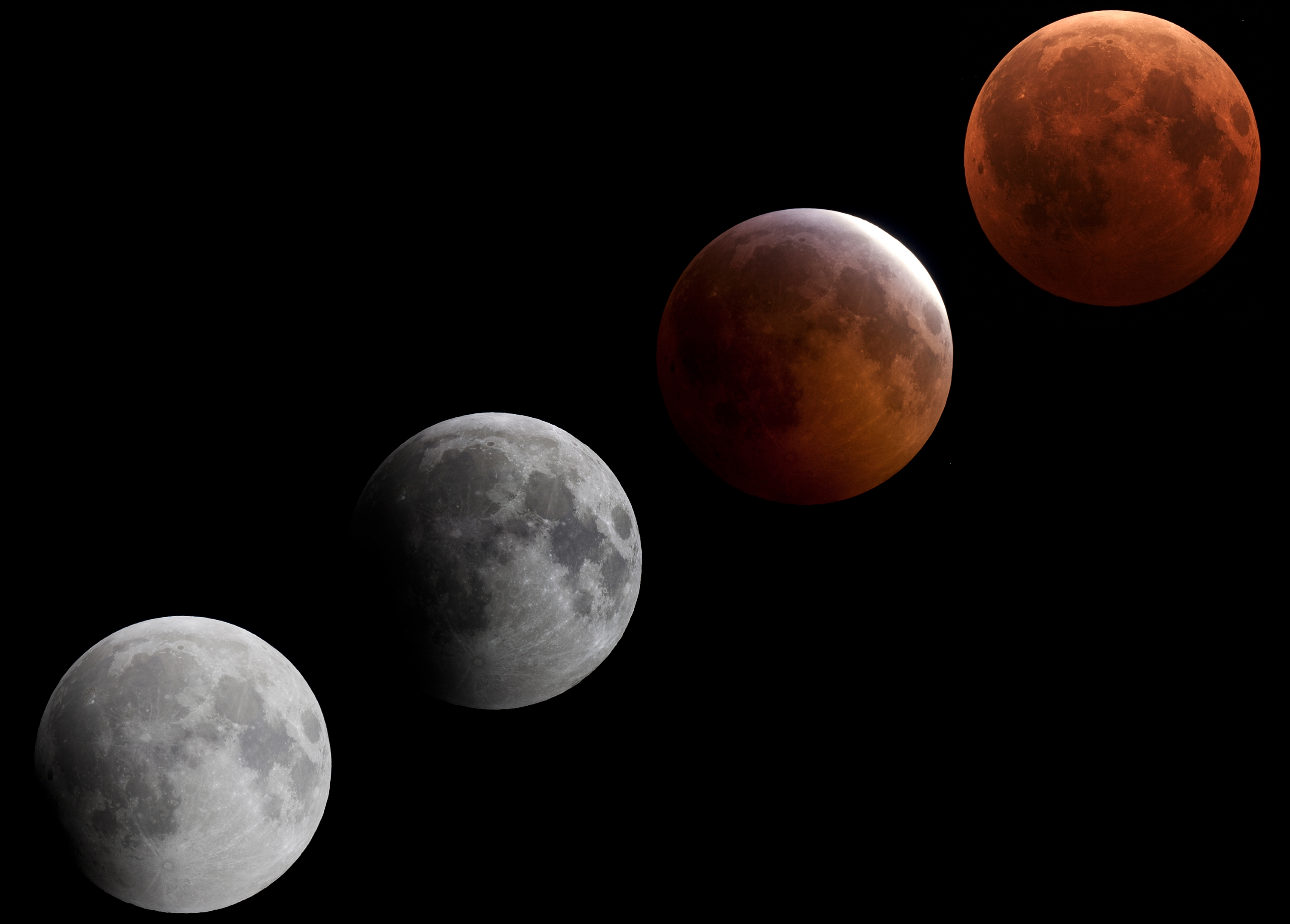The image features four distinct orbs, aligned diagonally from the bottom left to the top right against a pitch-black backdrop. The orbs, which resemble phases of the moon, transition in color and shading as they progress upwards. The first orb in the bottom left is white with gray patches, reminiscent of a full moon. Moving diagonally upwards, the second orb displays more shadowing while still maintaining its gray color scheme. The third orb introduces a reddish-orange hue, partially shadowed with a bright top, suggesting illumination from an external light source. The final orb in the top right is fully colored in a dark reddish-orange, devoid of shadows, presenting a complete transition. This alignment represents a visually captivating evolution, illustrating the changing phases of a moon-like object in a sequential manner across a seamless, one-dimensional plane.